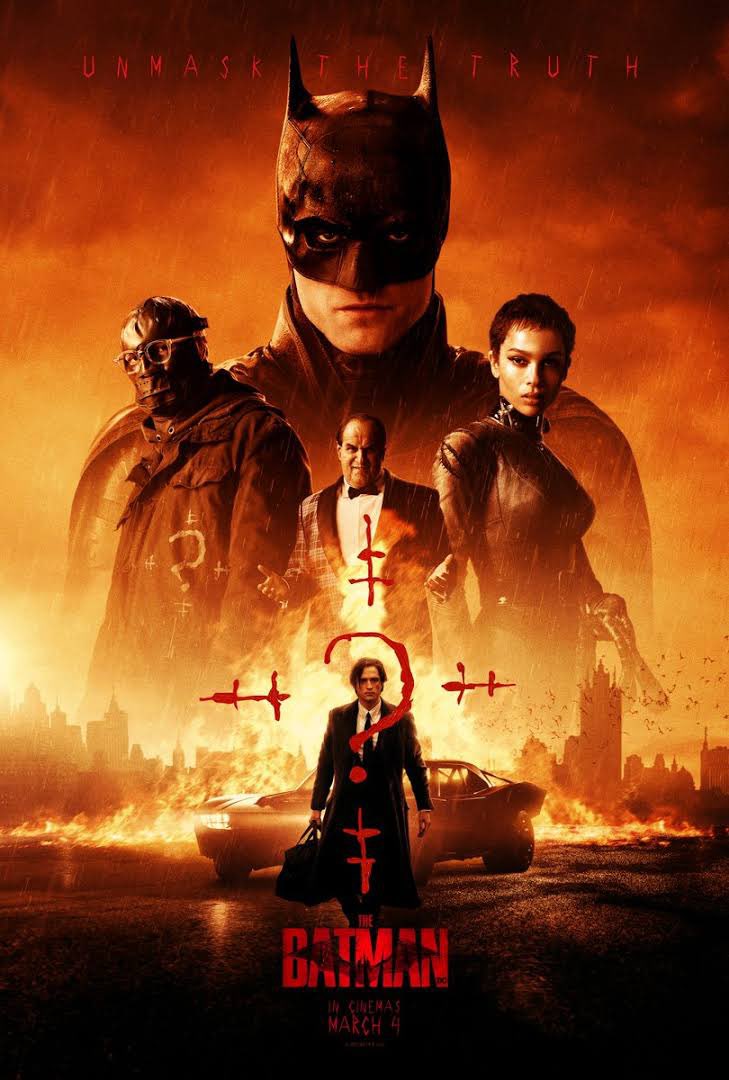This detailed movie poster for "The Batman" features a dramatic nighttime scene with a city engulfed in flames in the background. The sky glows ominously with dark red and orange hues, reinforced by heavy clouds and rising smoke. Amidst this chaotic backdrop, the faint silhouettes of tall buildings, the Batmobile, and fluttering bats are visible, alluding to a sense of unrest and danger. 

Dominating the foreground are the principal characters: Batman, centrally positioned in his signature black suit complete with mask, pointed ears, and cape; the Riddler, identifiable by his mask, glasses, and question mark insignia; the Penguin in his characteristic suit; and Catwoman in a tight bodysuit. Each character's head appears prominently, giving them an imposing presence over the fiery cityscape.

At the bottom of the poster stands Robert Pattinson, out of costume, representing Bruce Wayne. He is dressed in a black suit and carries a black briefcase, illustrating his dual identity. Above his head is a stylishly designed question mark, reinforcing the film's enigmatic and suspenseful theme. Encircling the scene is the tagline "Unmask the Truth," and beneath it, the title "The Batman" with the Bat logo and release date, "In Cinemas March 4th."